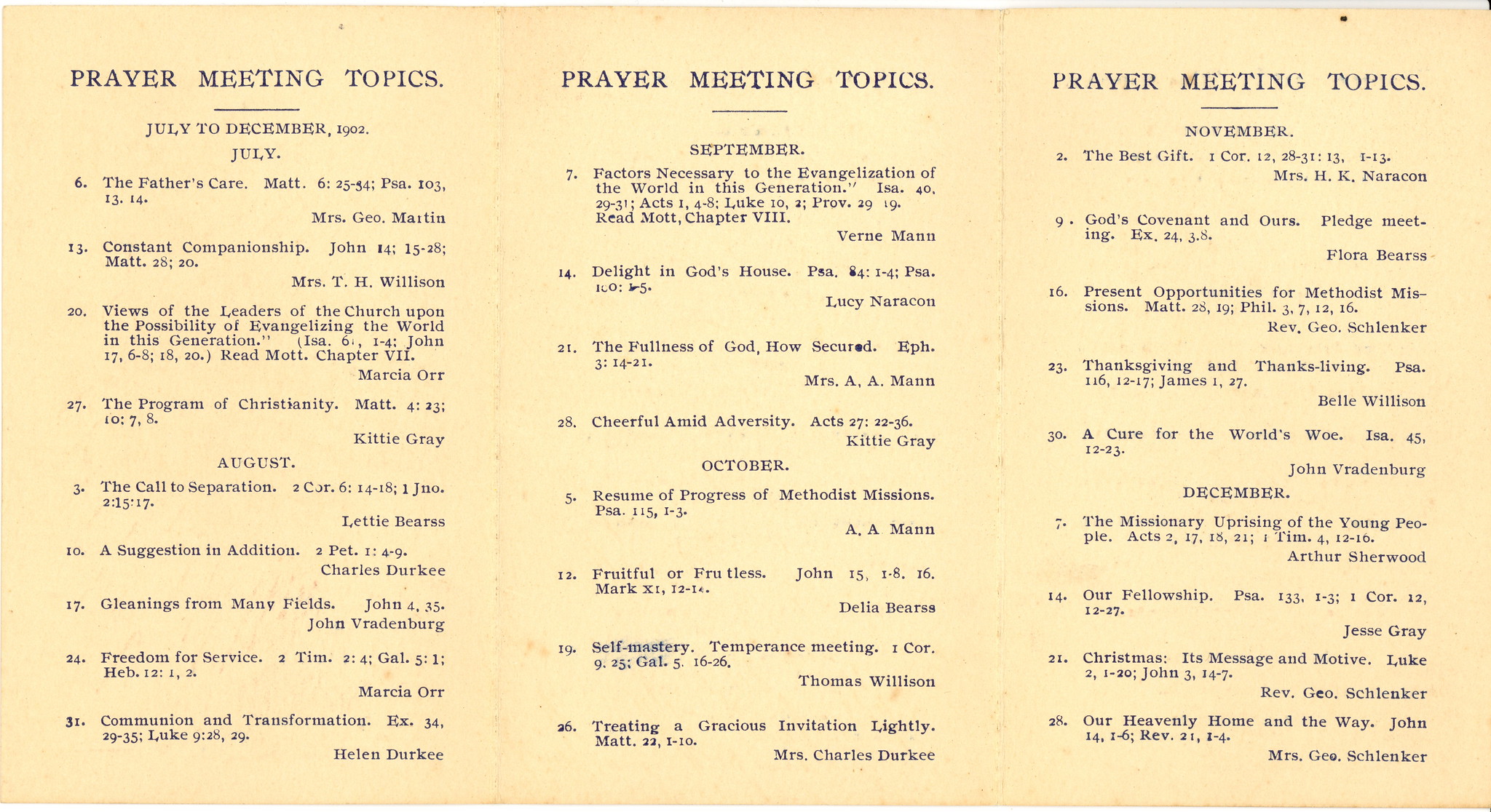The image depicts a trifold piece of yellow-hued cardstock paper listing prayer meeting topics, covering the period from July to December 1902. Each of the three sections is titled "Prayer Meeting Topics" at the top, with a clear underline. The left section details topics for July through August (with dates such as the 6th, 13th, 20th, and 27th of July), the middle section covers September to October, and the right section outlines November to December's schedule. Each entry includes a statement, a Bible passage reference, and a name, indicating who will be reading or leading each topic. The paper appears worn, showing individual fibers and a slight yellowish-brown discoloration, suggesting age and heavy use. The print is clean, with black text providing clear visibility despite the aged appearance of the paper.